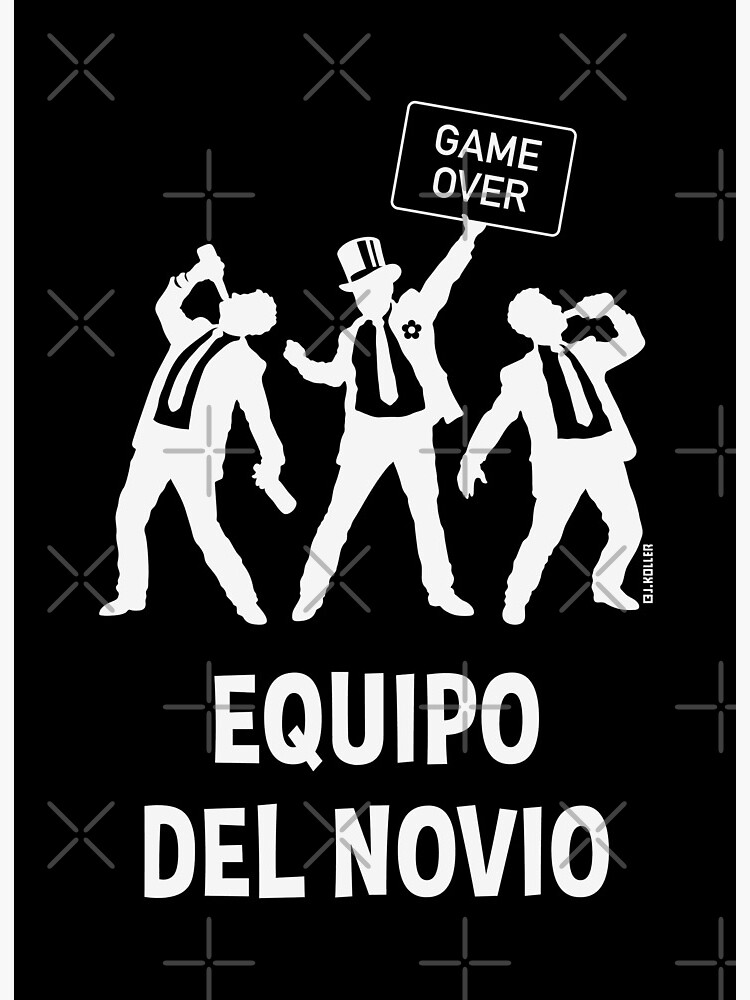The image is a vertically oriented poster set against a dark grey, almost black background, with intricate white elements. At the bottom, bold white text reads "Equipo del Novio," which translates to "Groom's Team." Overlaying the entire image is a repeating pattern of grey crosses and X's, resembling a watermark.

In the foreground, there are three male figures dressed in suits. The man on the left is depicted in a suit and tie, energetically drinking from a bottle while holding a second bottle in his other hand. On the right, another man, similarly attired, is also tilting a bottle back to drink, though he holds no additional bottle. Dominating the center is a man wearing a top hat and a flower pinned to his jacket; he stands out as he holds a sign proclaiming "Game Over." This central figure's top hat appears to be black and shiny, giving it a distinguished look. The name "J. Coller" is also visible, written vertically, suggesting the artist or creator of the piece.